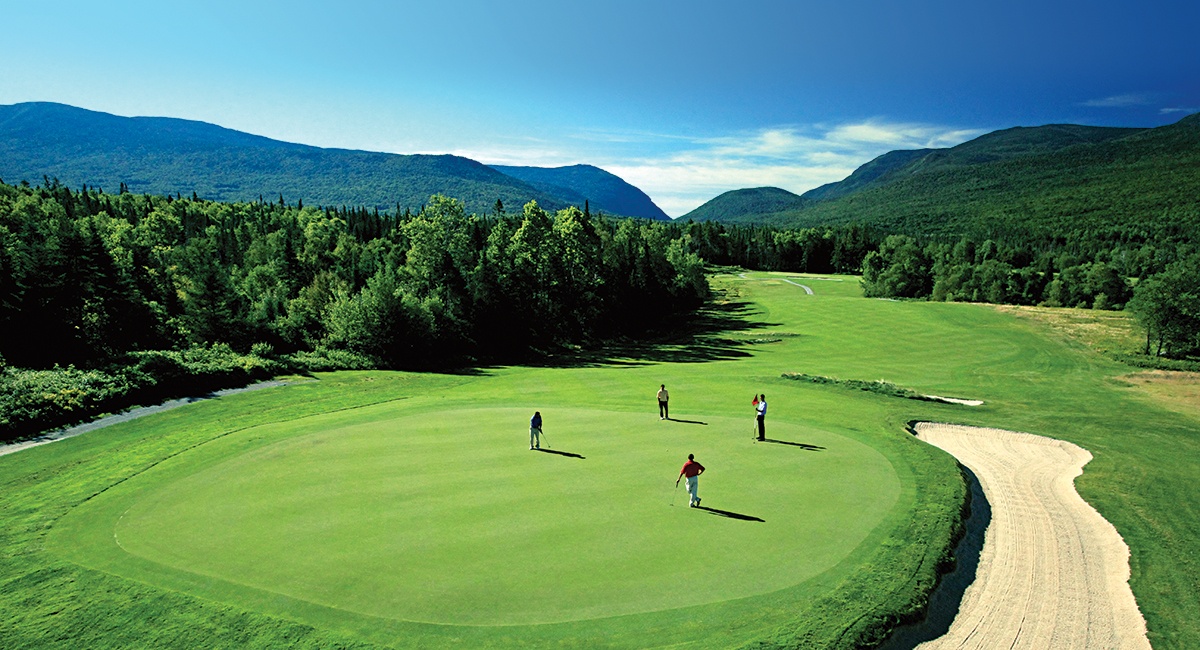The image captures a bright and picturesque aerial view of a golf course set against a backdrop of rolling, mountaintop scenery under a clear blue sky. In the center of the photo, four golfers stand on a smooth greenway, casting long shadows that suggest the photo was taken early in the day. One golfer, dressed in a short sleeve red shirt and white pants, stands near three others; one in a white shirt, and another in a dark shirt bent down with a golf club, preparing to hit a putt towards the hole where the flag is still up. Surrounding the greenway are lush, tall green trees, creating a forested tunnel effect around the course. To the right of the green lies an elongated sand bunker, and the fairway stretches lengthwise back toward the starting point, enhancing the depth of the scene. In the distance, the serene mountains complete the idyllic outdoor setting.